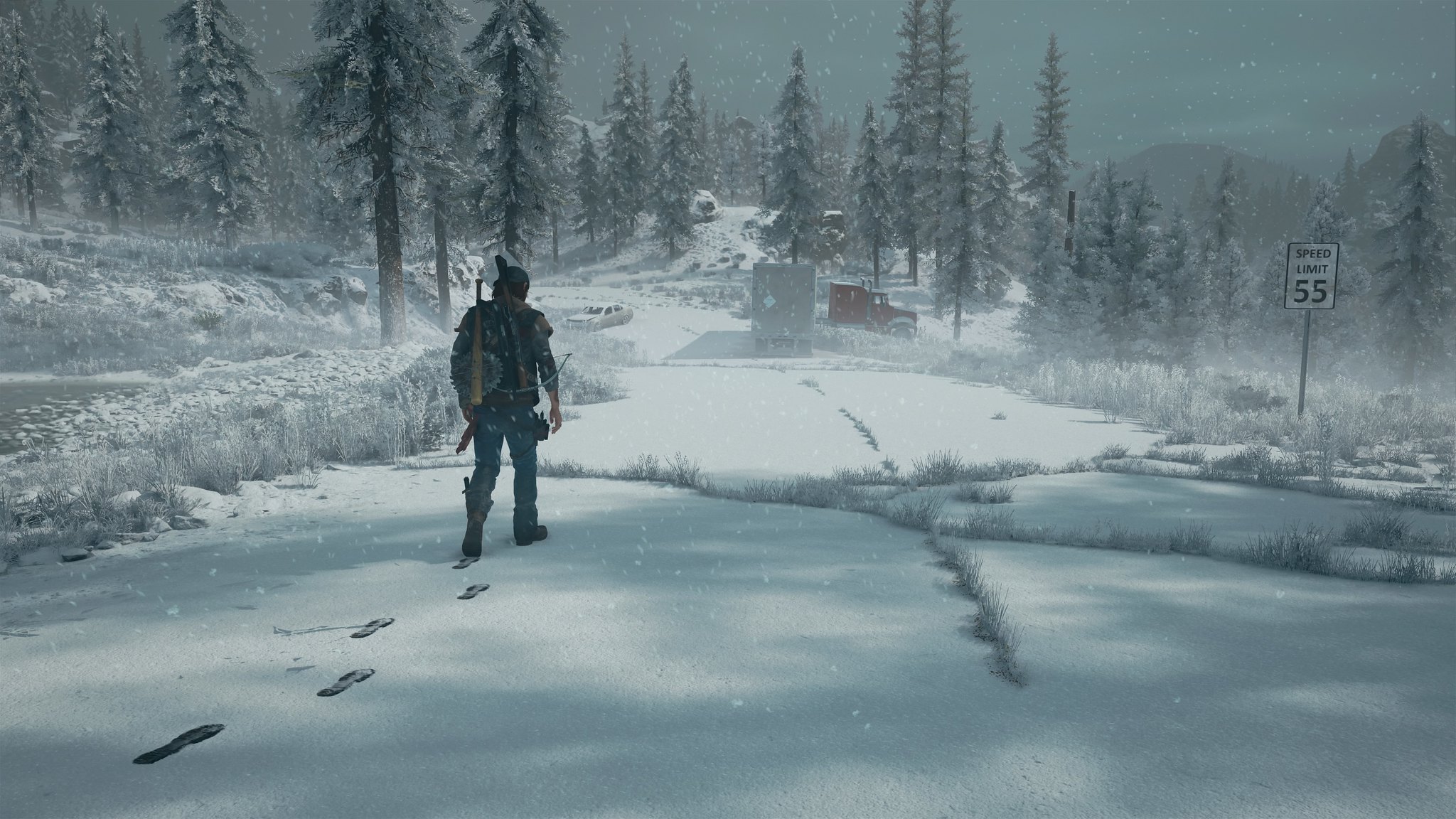The black-and-white image depicts a winter scene in a rural, northern climate. Snow covers the ground and blankets the pine trees in the background. A road, seemingly rarely used due to visible grass growing in the cracks, cuts through the landscape. Although the road looks desolate, a speed limit sign sets the limit at 55 miles per hour, creating a hint of inconsistency in the scene.

In the left foreground, a man wearing jeans and a hat but notably missing gloves, walks towards the camera, leaving clear footprints in the snow behind him. He is carrying several items on his back, possibly weapons and other garb, adding a curious element to his journey.

Further down the road, a semi-truck has slid off into a ditch, with the rig still on the road while the cab dangles off to the side. Nearby, a white station wagon appears to have veered off the road as well. Although it is snowing, the sky has a peculiar brightness to it, almost as if the sun is out. This, along with the meticulous detailing and minor inconsistencies like the lack of fresh tracks where the vehicles skidded off, raises questions about the reality of the image, suggesting it might be computer-generated.